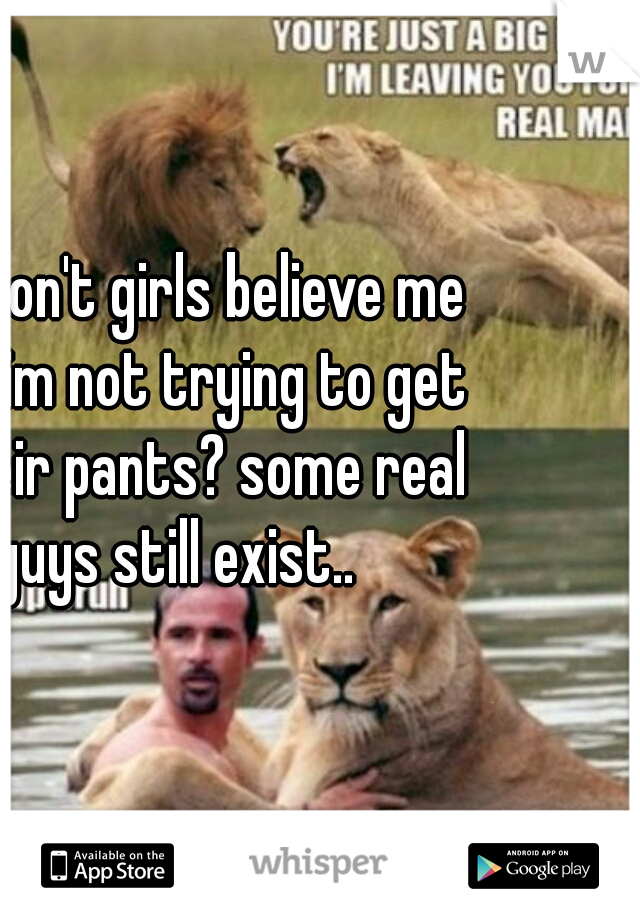The image appears to be a meme or advertisement for the app Whisper, available on the App Store and Google Play. The top right corner features the Whisper logo, a stylized "W" with a page fold. At the very bottom, centered, "Whisper" is written in grey letters. On the bottom left is the App Store logo for Apple, and on the bottom right, the Google Play Store logo for Android.

The meme is divided into two panels. The top panel shows a male lion and a growling lioness on grass. The visible text, in all caps white letters, reads: "YOU'RE JUST A BIG [CUT OFF TEXT]. I'M LEAVING YOU FOR A REAL MAN." The bottom panel features a shirtless man in the water, holding a calm lioness. The accompanying text, in white letters with a black outline, says: "DON'T GIRLS BELIEVE ME? I'M NOT TRYING TO GET IN YOUR PANTS. SOME REAL GUYS STILL EXIST." The imagery contrasts the aggressive lioness in the top panel with the serene scene involving a human and the lioness in the bottom panel, implying a message about genuine masculinity.